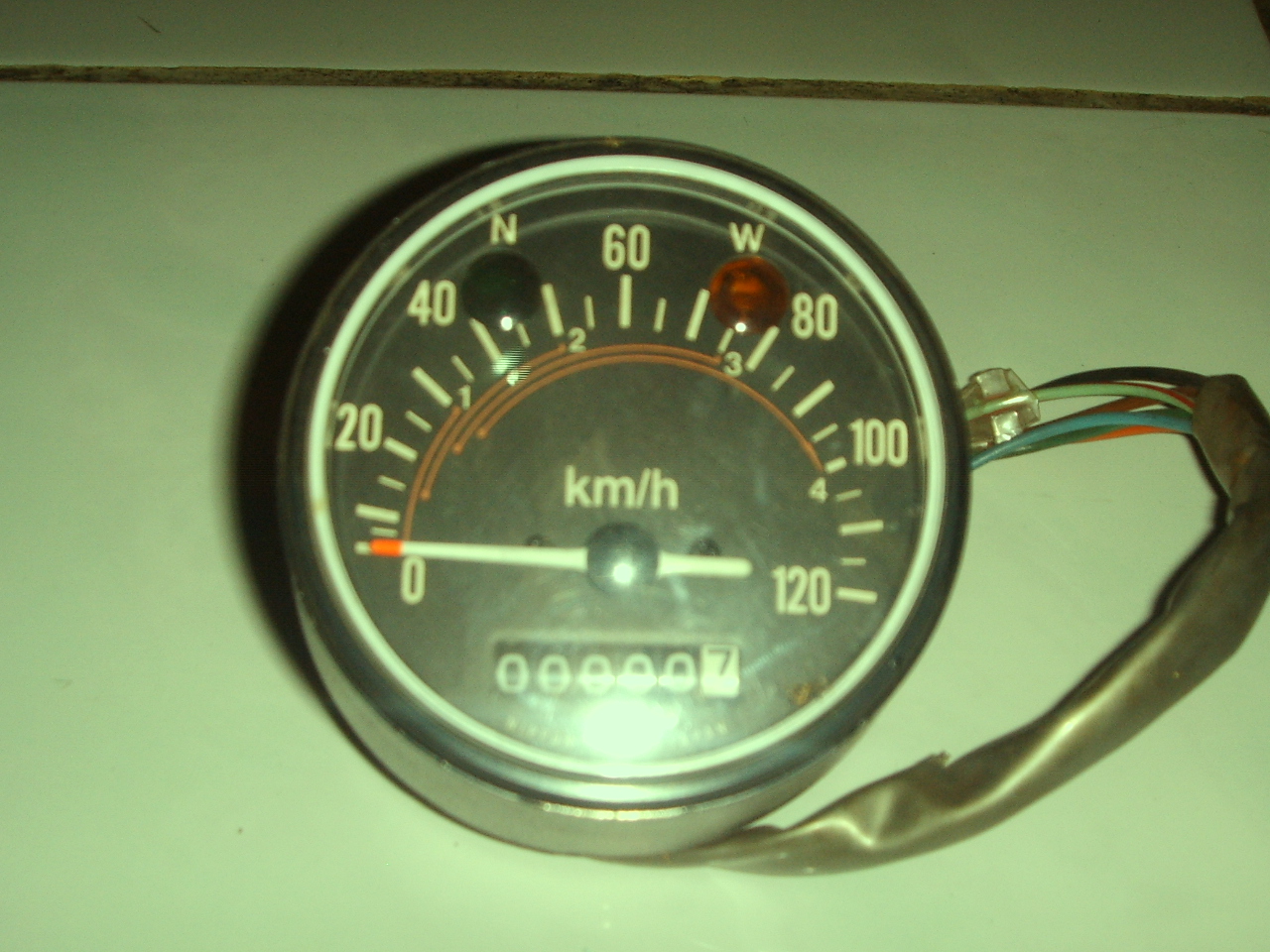The image depicts a close-up shot of a large square surface, likely a flooring tile, with a smooth sage green color. The tile is intersected by a brownish grout line, which shows signs of wear and reveals a tan hue beneath the surface. The background appears to be part of a sequence of similar tiles, indicating it is probably a floor.

Light and shadows are cast unevenly on the tile, creating variations in the shade and brightness of the green color. In the center of the image is a circular gauge. The gauge features a black outer rim, a white inner rim, and a black face. The gauge is marked with white dashed lines along with numbers at intervals of 20, 40, 60, 80, and 100, with smaller lines in between.

Additional details on the gauge include numbers 1 through 4, an 'N' at the top with a black circle below it, and a 'W' with a red circle below it. An arch of orange lines is also present. The gauge measures speed in kilometers per hour and currently points to zero. At the bottom of the gauge, there is a counter reading "000007."